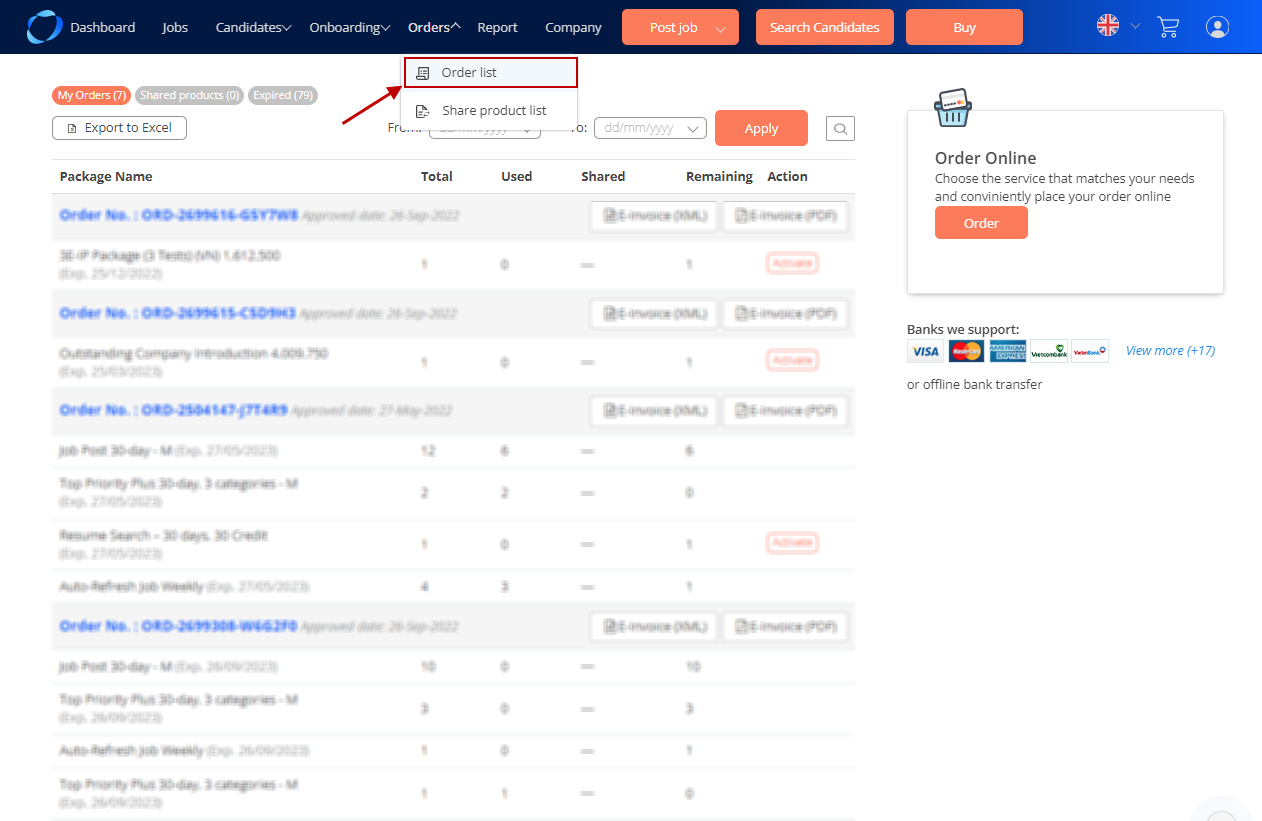The image showcases a comprehensive job recruitment website interface. At the top, the navigation bar prominently features various sections including Dashboard, Jobs, Candidates, Onboarding, Orders, Report, and Company. Below the navigation bar, three vibrant orange buttons stand out, labeled "Post Job," "Search Candidates," and "Buy," indicating functionalities for job postings, candidate searches, and purchases respectively.

Further down, there is an option to "Export to Excel" and to "Order a List," providing users with practical data management and ordering capabilities. The central portion of the page is dominated by four blue-highlighted items, listed sequentially by their order numbers, which are intentionally blurred out for privacy. These items are arranged in a table format with columns titled Package Name, Total, Used, Shared, Remaining, and Action, though the specific details within these columns are also blurred.

In the bottom right corner, a small box invites users to "Order Online," encouraging them to choose the service that best meets their needs and conveniently place their order online. Directly below this box is an "Order" button, ready to be clicked. The website also displays available payment methods underneath the order section, ensuring users understand their payment options.

This detailed interface suggests strong functionalities oriented toward both hiring processes and procurement actions, enhancing user convenience and operational efficiency.